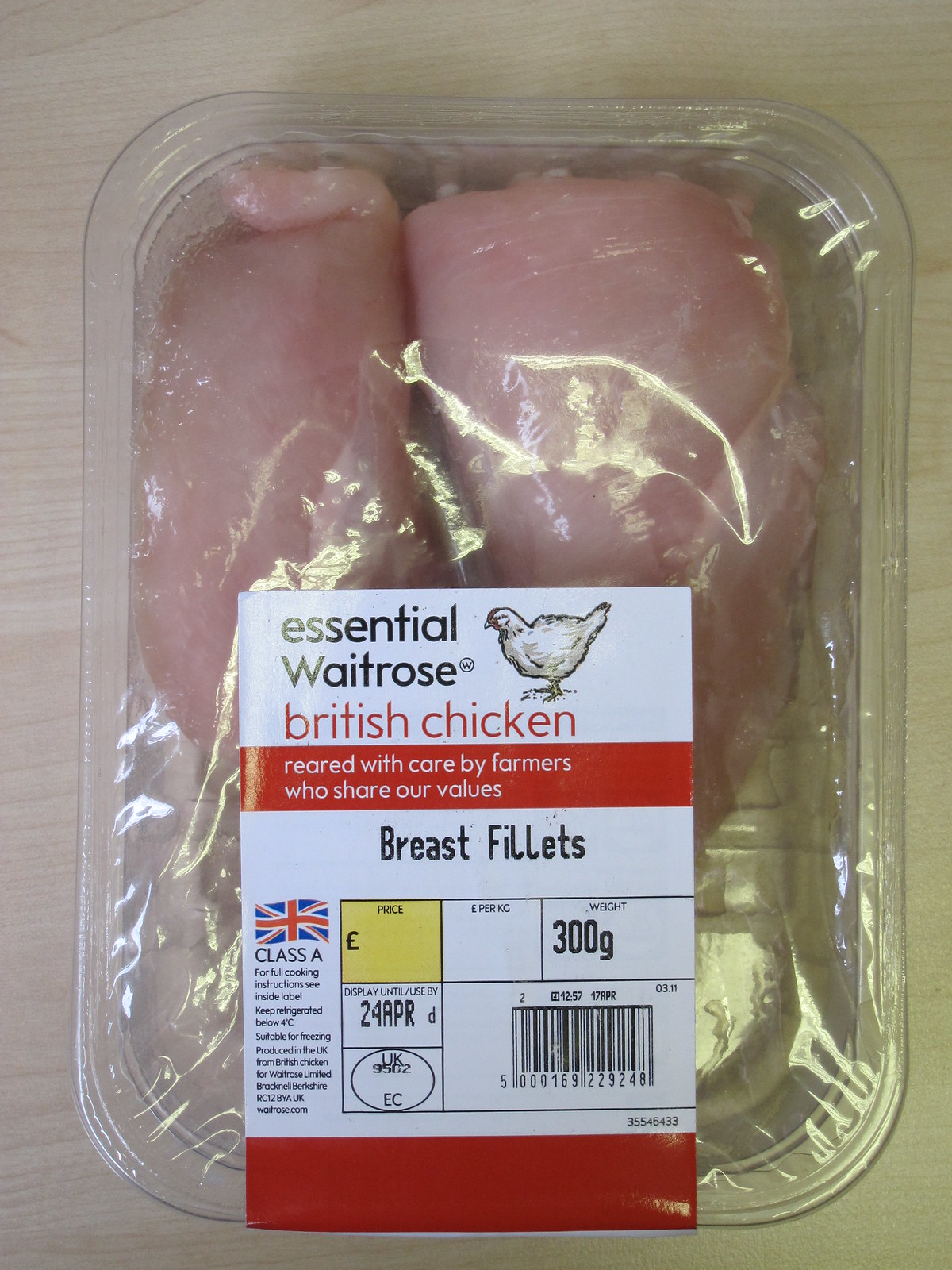This detailed, full-color overhead photograph captures a clear plastic package containing two chicken breast fillets. The package features a prominently displayed white label adorned with black and red text. At the top, the label reads "Central Wacross" alongside a drawing of a chicken. It further states, in bold red letters, "British Chicken, Reared with Care by Farmers Who Share Our Values," emphasizing the product's quality and ethical standards. The packaging also includes the Union Jack flag, indicative of its British origin, and identifies the chicken as "Class A." Additional details include the weight of the chicken, 300 grams, and a sell-by date of April 24th, 2024. While the label provides comprehensive information, notably, it does not list a price. The package is set against a brown table, adding a rustic backdrop to the image.